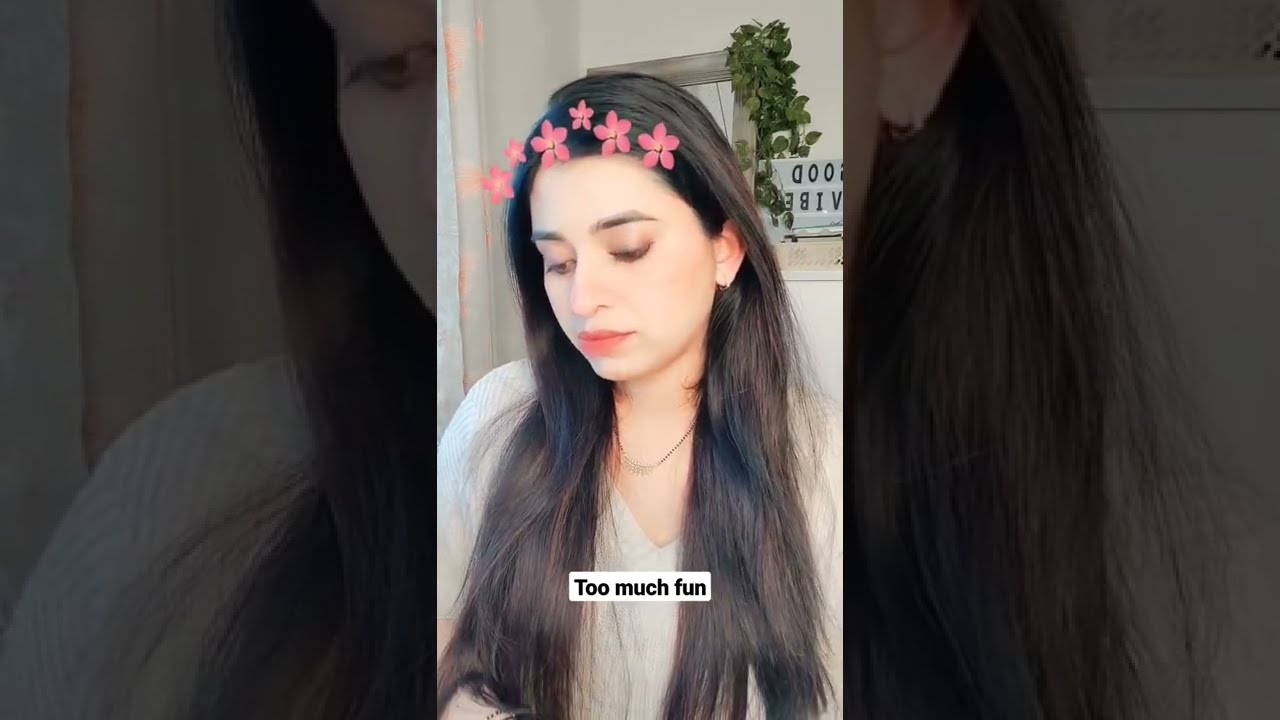In this indoor image, a woman with long, dark brown hair adorned with pink flowers is centrally positioned, taking up most of the frame. She is wearing a necklace and a beige or white sweater and is looking slightly downwards to her left. The scene features various background elements including a mirror, a green plant, a white door, and a sign reading "good vibes." Notably, there is a text overlay at the bottom of the image that says "too much fun" in black letters within a white bracket. This photo, captured with a filter adding flowers to her hair, appears to be a screenshot from a mobile app like TikTok or Instagram Live.